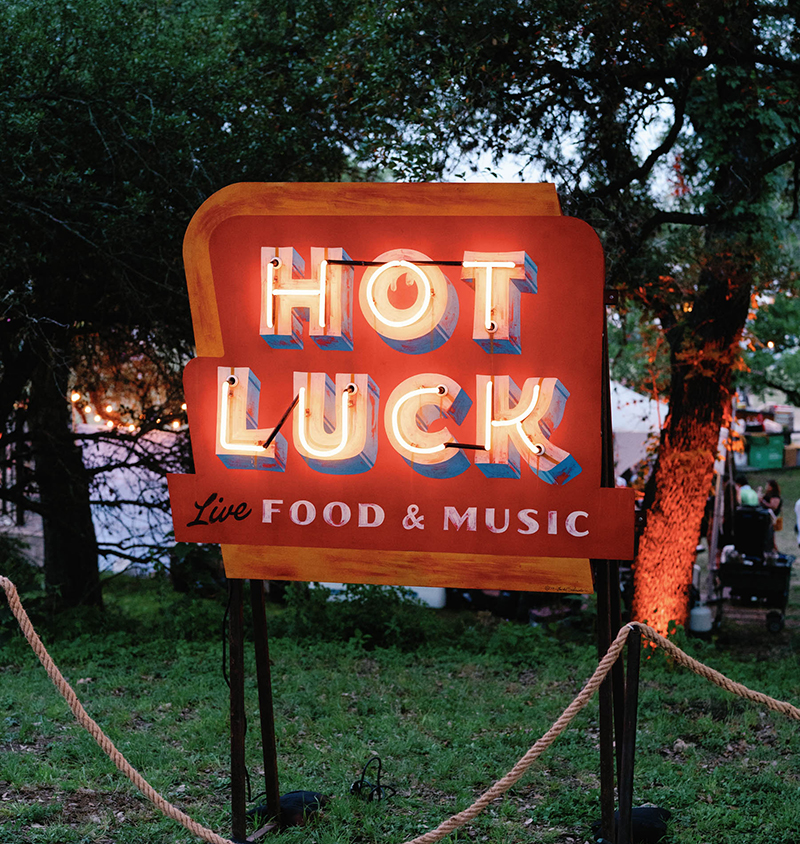Square in shape, this vibrant color photograph captures the lively atmosphere of a festival. Dominated by a striking neon sign that reads "Hot Luck Live Food and Music" in artistic text, the image is rich with detail. The neon sign, standing on metal poles, glows brightly against the backdrop, enticing attendees and passersby alike. A light brown rope, reminiscent of those used at galas or gatherings, stretches in front of the sign, guiding the flow of the crowd.

Behind the sign, various tents are scattered across the background, hinting at the festival's diverse offerings. A tree adorned with red highlights encroaches from the right, adding a splash of natural color to the scene. Additional trees dot the landscape, blending the festive human activity with natural beauty.

In the green lawn foreground, people are visible, some seated and possibly enjoying a meal. This energetic snapshot encapsulates the essence of a festival celebrating food, music, and conviviality.